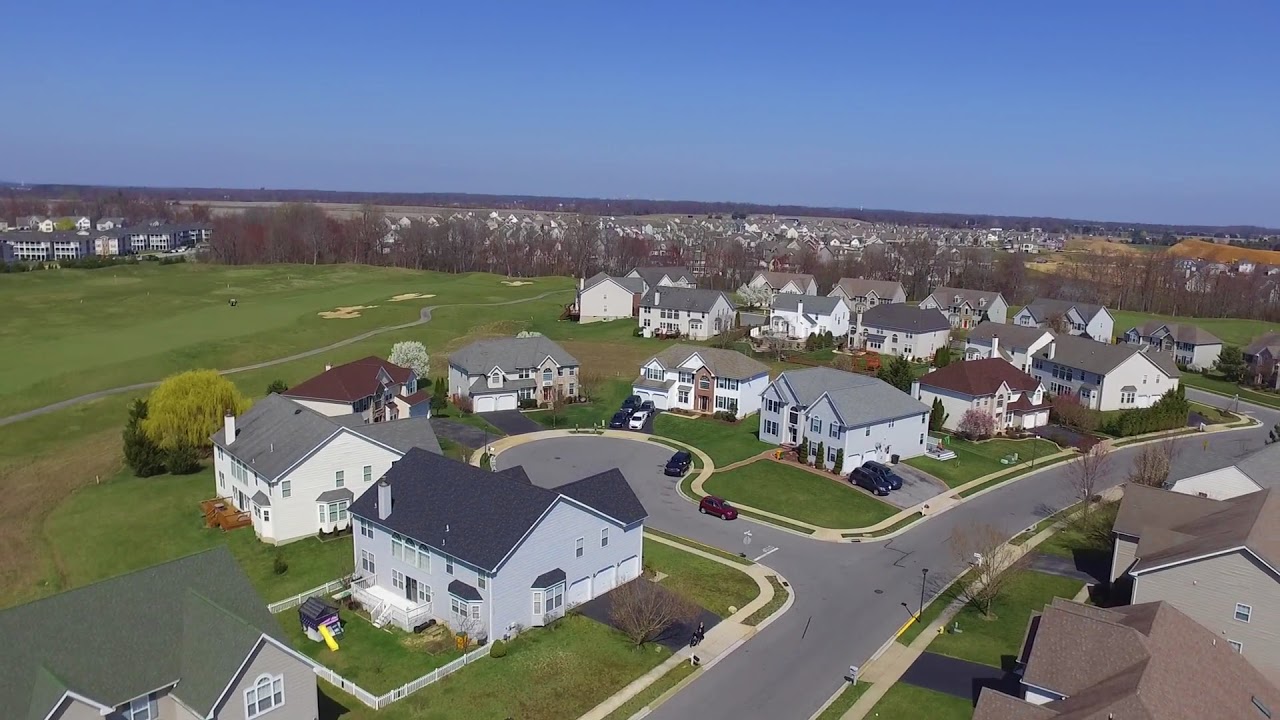Aerial image of a serene neighborhood filled with two-story, ranch-style houses nestled among lush, short-cut green lawns. The roofs of the houses vary from shades of blue, gray, and green to a standout red one. The streets are paved with light gray asphalt, featuring a curving street that leads into a cul-de-sac towards the center of the image. Prominent internal garages can be seen, with most houses having two or three-car spaces. To the far left, there is a meticulously maintained golf course, identifiable by its green fairways and sand traps. The backdrop includes a series of trees with dark amber leaves, creating a striking contrast against the clear, blue sky above. Beyond these trees, more houses spread out towards the horizon, interspersed with additional tree lines, stretching across a notably flat landscape.